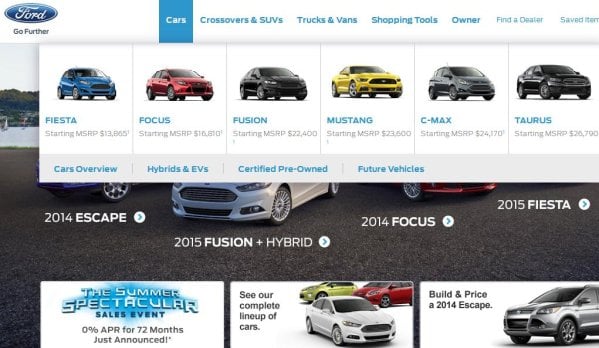The image showcases a section of the Ford Motor Company website, prominently featuring the iconic blue oval with the white Ford logo. Directly beneath the logo is the tagline "Go Further." The website interface appears to be divided into various categories such as Cars, Crossovers & SUVs, Trucks & Vans, Shopping Tools, Owner, Find a Dealer, Saved, Cart, and Edit. The list of vehicles highlighted includes models like the Fiesta, Focus, Fusion, Mustang, C-Max, and Taurus, along with sections for Cars Overview, Hybrids and EVs, Certified Pre-Owned, and Future Vehicles. These vehicle names are accompanied by corresponding images displayed against a white background.

In the pop-up at the bottom of the image, several car models are mentioned: the 2014 Escape, the 2015 Fusion plus Hybrid, the 2014 Focus, and the 2015 Fiesta. The bottom of the webpage prominently features the announcement of the Summer Spectacular Sales Event, advertising a 0% APR for 72 months. This section encourages viewers to explore the complete lineup of cars, with images of three vehicles (gold, red, and white) provided for reference. In the bottom right corner of the webpage, an option to "Build and price a 2014 Escape" is available.